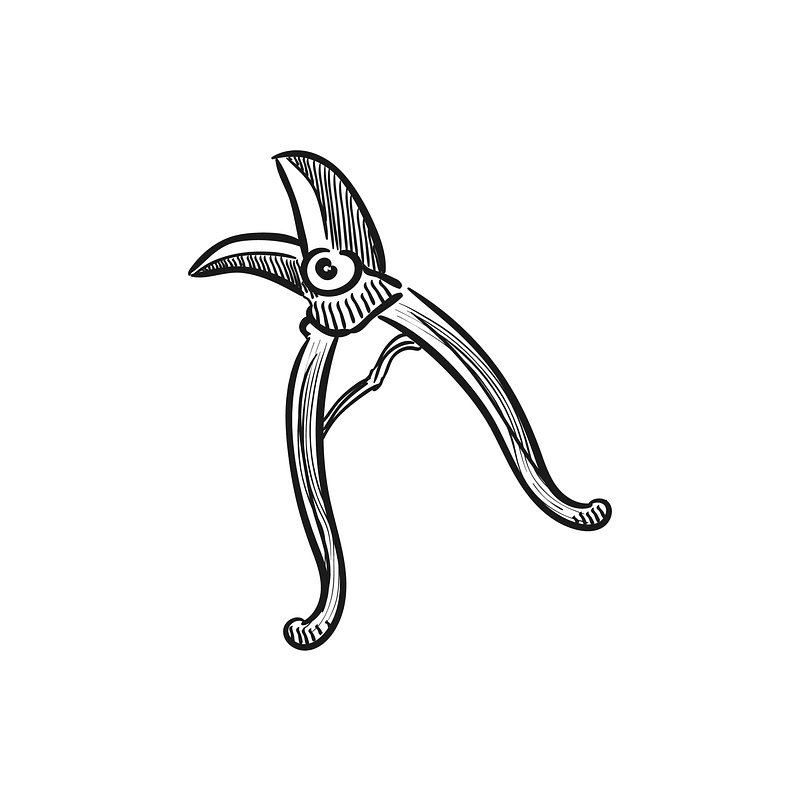The image depicts a detailed, cartoon-style pair of secateurs, a specialized gardening tool known for its curved cutting blades, similar to a parrot's beak. These blades are stubbier and fatter than typical scissors, with the top blade being noticeably wider than the bottom. The secateurs feature a set of curved handles that resemble those of pliers, which, when squeezed together, activate the linkage near the rivet, bringing the blades together to make a cut. The entire sketch is rendered with a black outline and rough shading to fill in the details of the blades and handles. The handles themselves taper slightly at the ends and curve gently to finish with a small nub. The secateurs are illustrated from a side view against a white background, emphasizing the large hinge between the blades and the connection at the handles. The drawing is done in pencil, with noticeable shadowing and black lines adding depth and texture to the image.